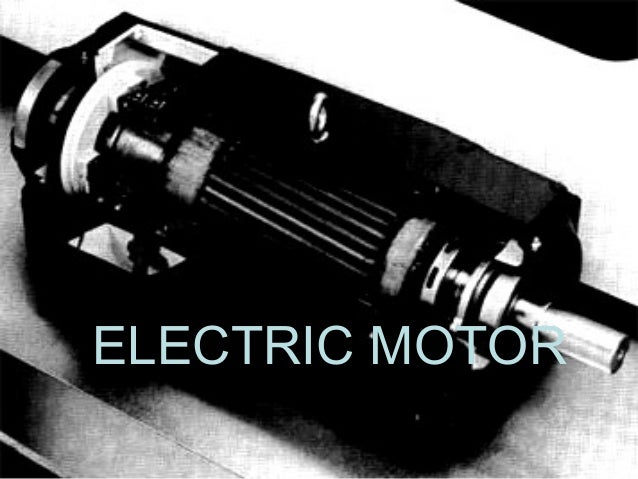This is an old black-and-white photograph depicting an electric motor, as indicated by the label "electric motor" centered along the bottom to middle portion of the image. The motor itself is predominantly dark in color, with shiny silver ends. On the right side, a silver handle is visible, while the left side features a silver turning piece or gear. The apparatus appears to be long and cylindrical, resembling a gear or part of an engine. The motor is adorned with long rivets and a noticeable casing that encloses various parts. This casing is elevated on a surface, which seems to be a lighter color and possibly soft, suggesting it might be cloth material. The surface below the cloth appears to be reflective or metallic. The background on the upper right side of the image is mostly white with a solid black corner, but these details are quite muted given the black-and-white nature of the photograph.